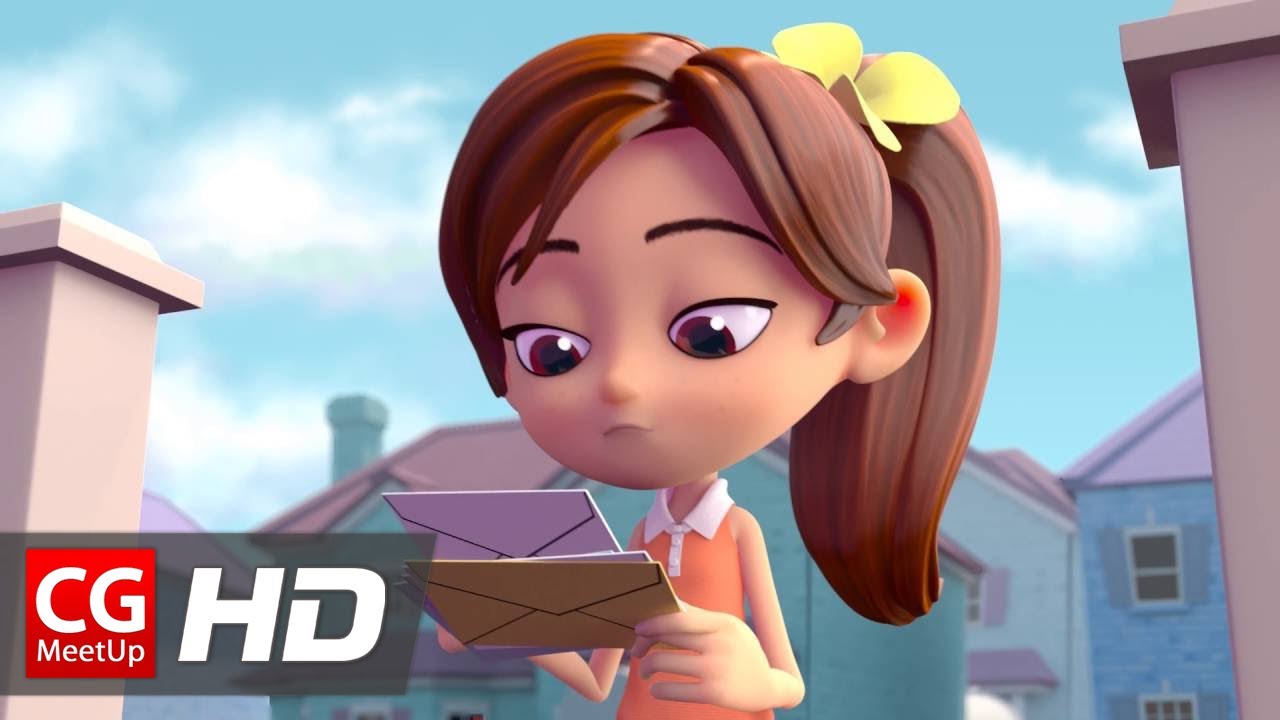In this 3D rendered cartoon image, a young girl, rendered in a simple yet charming style, stands outside with a collection of envelopes in her hands. She appears to be sorting through her mail, her hand held straight as she examines one of the envelopes. The girl has brown hair tied back into a ponytail, adorned with a large yellow flower at the hair tie. She's wearing a peach or coral tank top with a distinctive white collar, an outfit that seems designed to appeal to children. Behind her is a quaint town scene, with houses and possibly fence posts flanking her on either side, adding to the suburban ambiance of the image. The girl’s features include a notably small neck and a relatively large head, emphasizing the cartoonish style. In the bottom left corner of the image, the logo "CG Meetup HD" signifies the likely source or theme of this digital artwork.